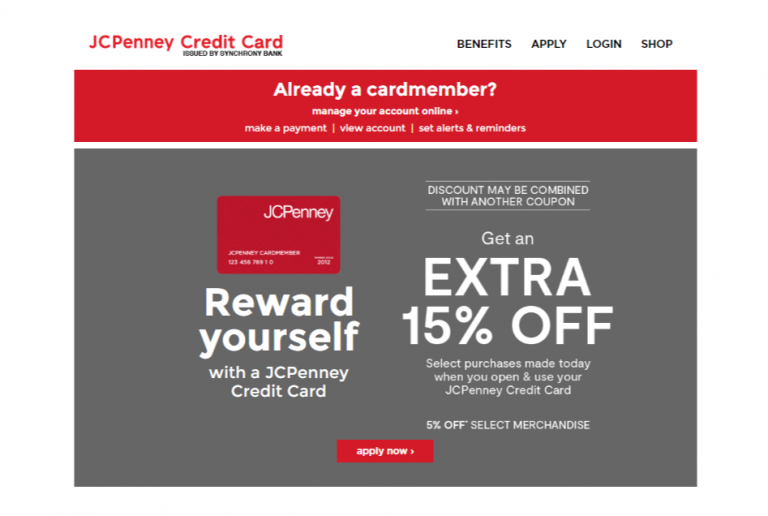The image features a promotional layout for a JC Penney Credit Card with an organized design on a varied background. The upper portion of the image is filled with a white background. Along the left-hand side of this white space, "JC Penney Credit Card Issued by Synchrony Bank" is prominently displayed in larger black and red text, with the latter in bold for emphasis.

Beneath this, smaller black text categorizes navigation options into four tabs: "Benefits," "Apply," "Login," and "Shop." Adjacent to it, there's a small red rectangle featuring a series of white text instructions including "Already a Card Member," "Manage Your Account Online," "Make a Payment," "View Account," and "Set Alerts and Reminders."

The remaining area of the image transitions into a grey background. On the left side, a red representation of a JC Penney Credit Card is prominently displayed with the statement "Reward Yourself with a JC Penney Credit Card" in white, positioned directly underneath the card image.

On the right side of the grey section, a series of promotional benefits is listed in bold white text: "Discount May Be Combined with Another Coupon," followed by "Get an Extra 15% Off Select Purchases Made Today When You Open and Use Your JC Penney Credit Card." Additionally, an offer of "5% Off Select Merchandise" is prominently highlighted.

Towards the bottom center of the image, a bright red rectangular button with striking white text invites users to "Apply Now" for the credit card.

This detailed layout combines clean, clear text and strategic use of color to effectively communicate the benefits and actions related to the JC Penney Credit Card.